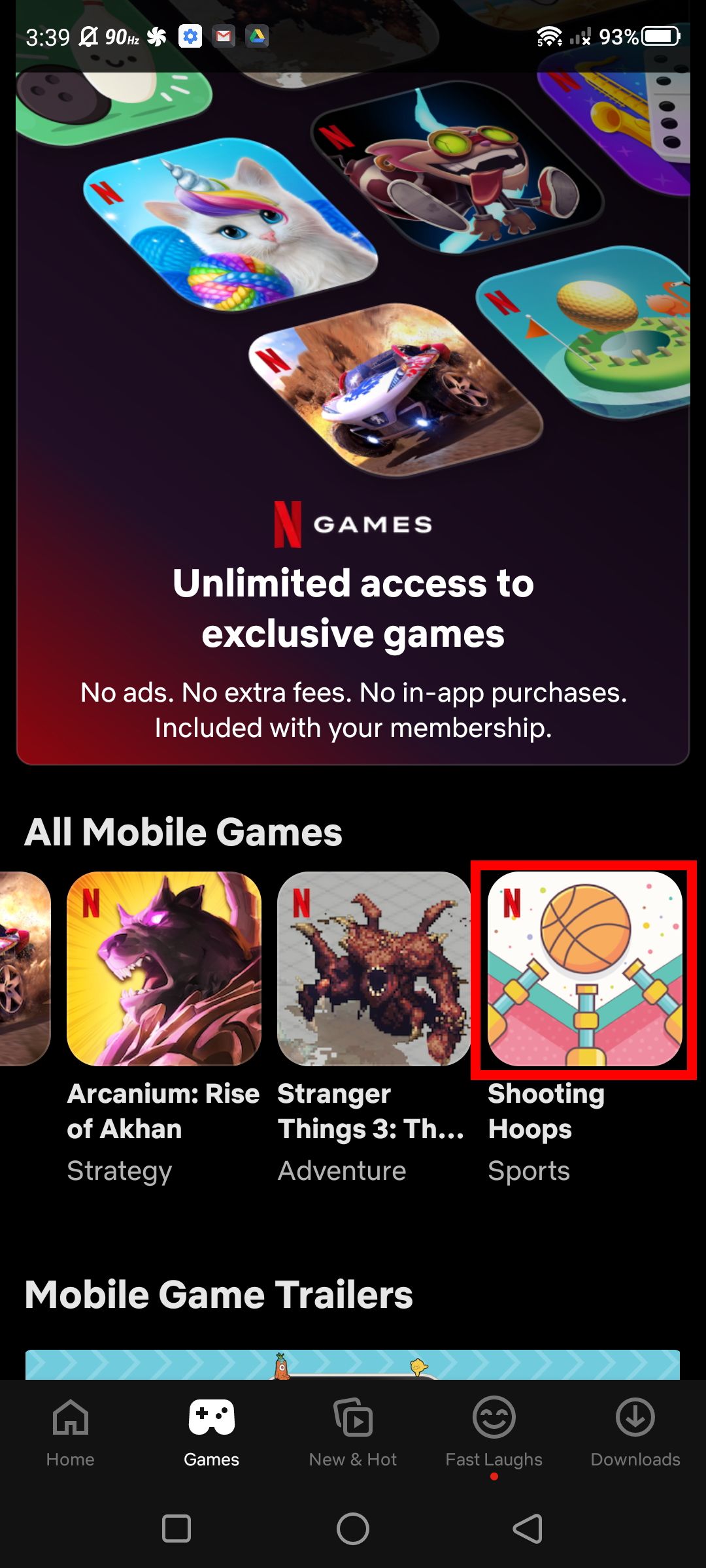Screenshot from a mobile device displaying the Netflix Games interface. In the upper left and right corners, various standard icons indicative of a cell phone's status can be seen. Dominating the screen is a section from Netflix Games, prominently featuring the brand's signature red 'N' logo in the top left corner of several app thumbnails. These thumbnails are aligned horizontally, depicting different game options.

At the top center of the screen, the Netflix Games logo is displayed, accompanied by the text "Games" in white font on a red background. Below this, a message reads, "Unlimited access to exclusive games," also in white font and center justified. Further down, a smaller, yet still center-justified section of text details, "No ads, no extra fees, no in-app purchases. Included with your membership."

Beneath these introductory texts is a horizontal scrolling bar showcasing available mobile games. The first visible game is "Arcanium: Rise of Arcan." Following it is "Stranger Things 3," demonstrating the diverse range of gaming options offered by Netflix.